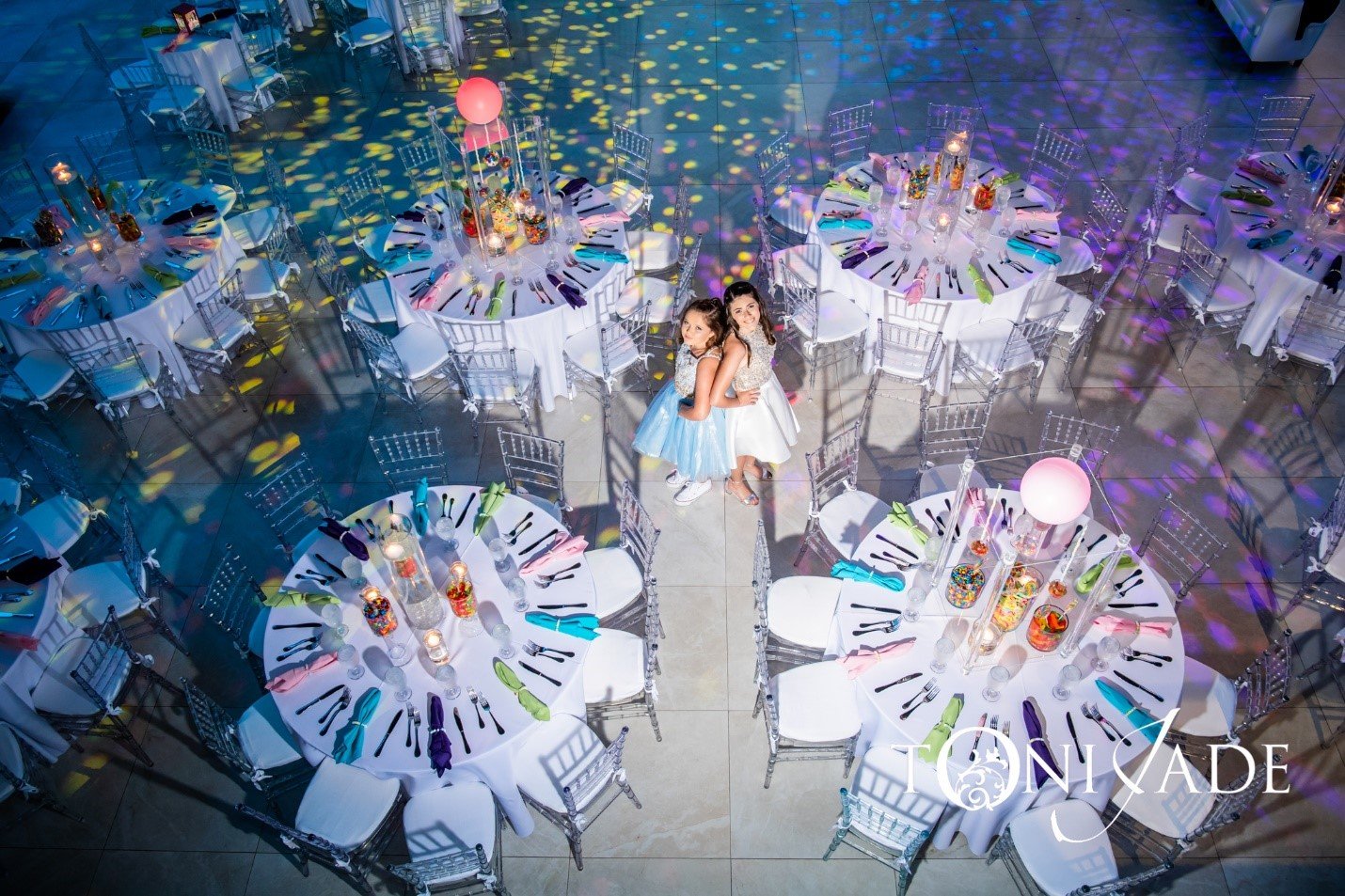In this enchanting overhead photo taken in an indoor event space, two little girls stand back-to-back in the center of the image, poised in their charming party dresses—one adorned in blue and the other in white. Both girls, with their dark hair and hands confidently resting on their hips, gaze upward at the camera. Surrounding them are four round tables draped in pristine white tablecloths, hosting neatly arranged settings with silverware and vividly colorful napkins in shades of pink, blue, purple, and green. Each table is further decorated with playful balloon centerpieces, adding a festive touch. The shiny white floor below gleams under the event lighting, and a sprinkling of confetti is visible, amplifying the celebratory atmosphere of what appears to be a delightful birthday party. This horizontally cropped image, complete with a watermark in the bottom right corner bearing the name "Toni Jade," captures a moment of joy and elegance.